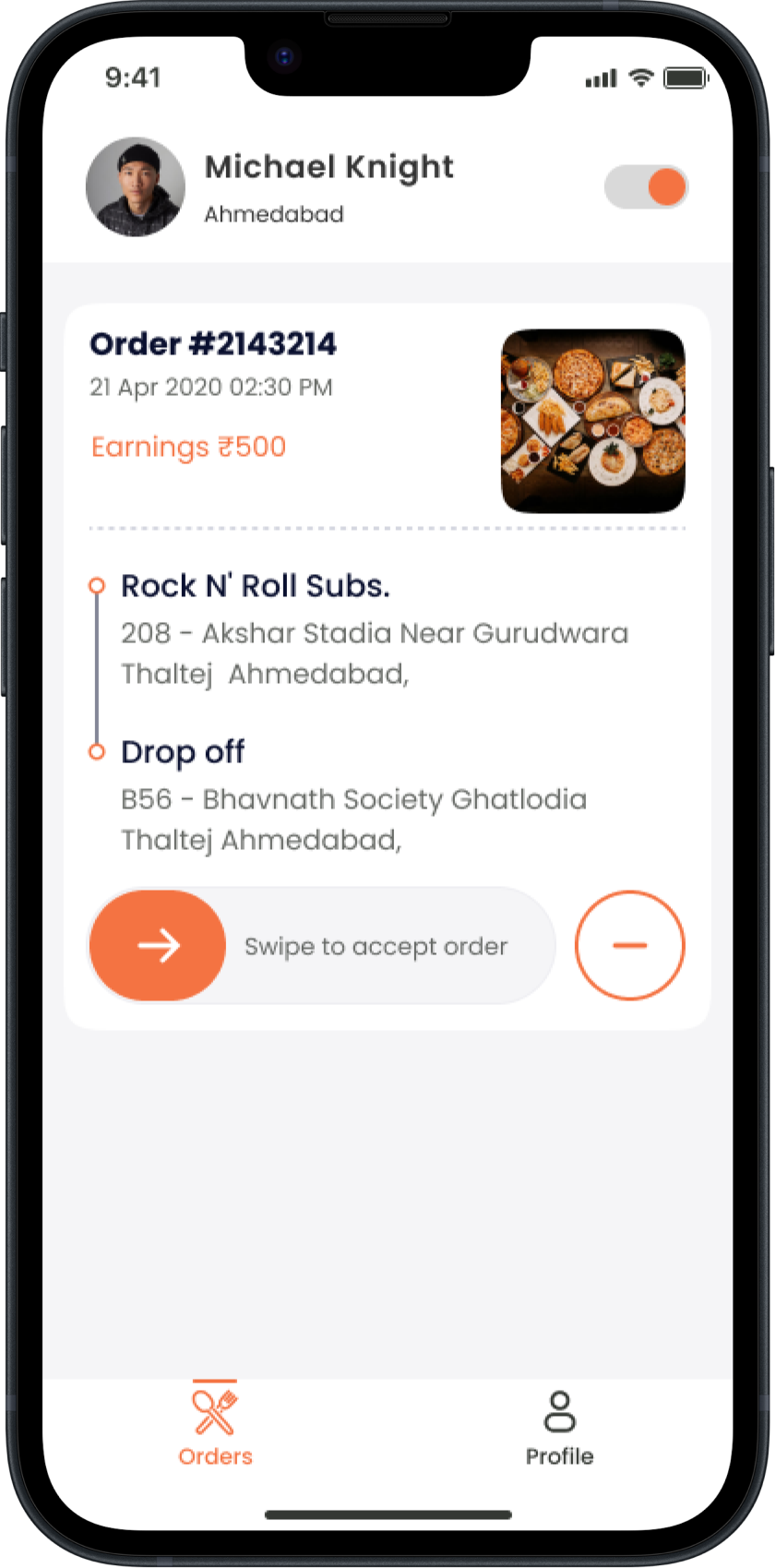**Caption:**

The image displays the interface of a smartphone screen captured at precisely 9:41 AM, as indicated by the white text at the top left corner. Adjacent to the time, there's a series of status icons including a middle speaker symbol, a 4G signal bar, a full WiFi signal bar, and a fully charged battery icon, all lying against the black break of the phone’s interface.

Just below this top bar is a dark blue border featuring a circular black and white profile picture of a man named Jackson, spelled "J-A-X-S-L-A-N-N-E," located on the left. Directly beneath his picture, his location is listed as "Spain," and to the lower right, it is labeled "Top Story." An active, yet background-colored, selectable widget nodule is visible here.

The main section of the screen displays a summary of an order, designated as Order Number 214204. The order was placed on April 22nd at 2:30 PM. The earnings amount to $500, and the current item featured is a cheeseburger priced at $79. A large image of a cheeseburger is prominently displayed below this information. Additional details reference "Dave Dijon" and a figure "9610," though it's unclear if they relate directly to the item.

Below the cheeseburger image, the text reads "Drop-off for ABN." Extending from the bottom are two actionable buttons: on the left, an arrow suggests swiping right to accept the order, indicated by "Swipe right to accept." On the right is a dark blue circle containing a minus symbol, offering a different action.